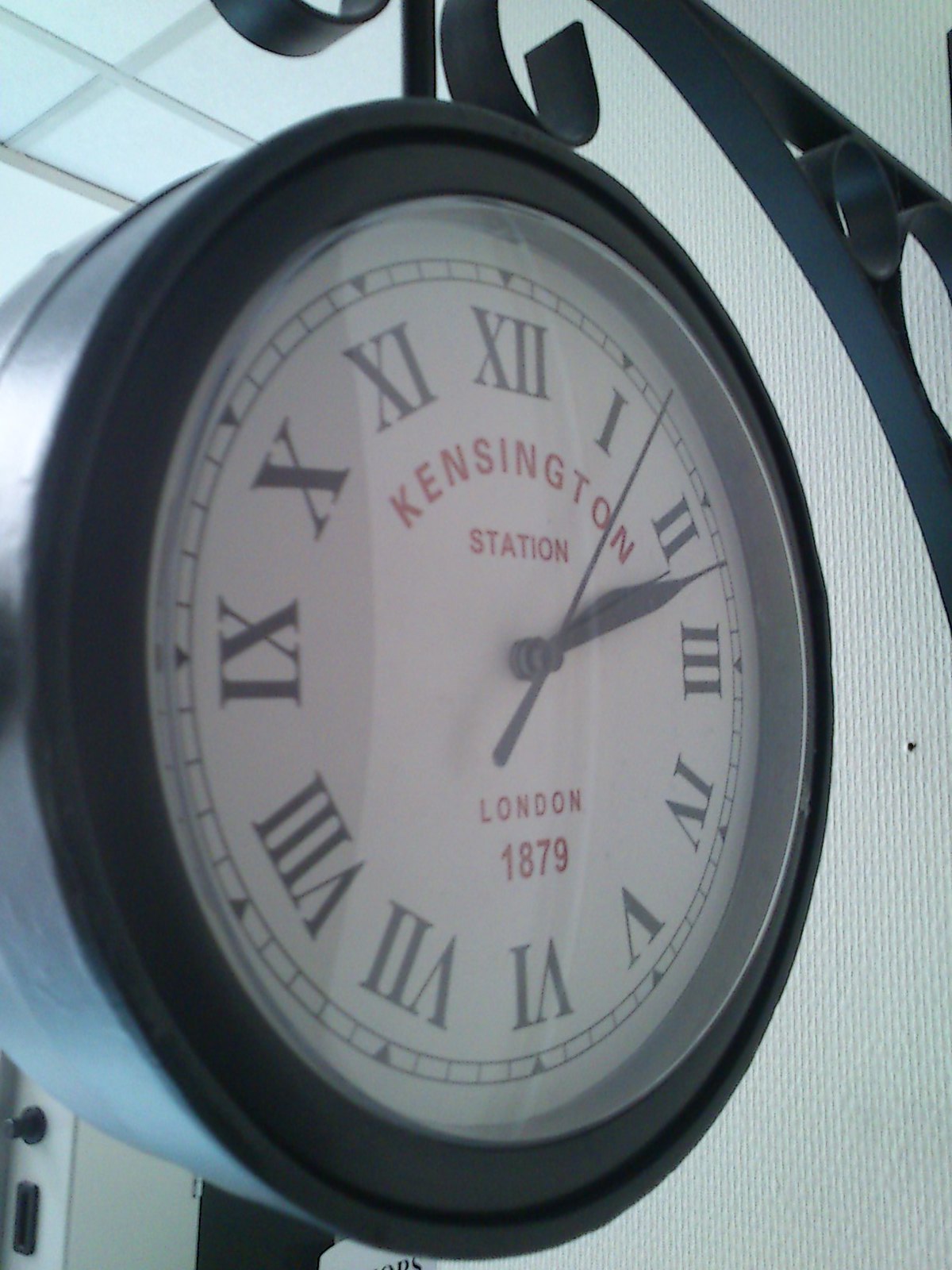A striking black clock with an elongated back is prominently displayed, hanging on a sturdy support. The setting is an indoor environment, as evidenced by a white drop ceiling and a textured white wall adorned with vertical lines. The clock's face features Roman numerals, each elegantly punctuated by downward-pointing triangles. The text "Kensington Station" stands out in red at the center, while the inscriptions "London 1879" are subtly positioned beneath the hands, which are also black. The background reveals a door fitted with a handle, a doorknob, and a classic keyhole, adding a touch of vintage charm to the scene.